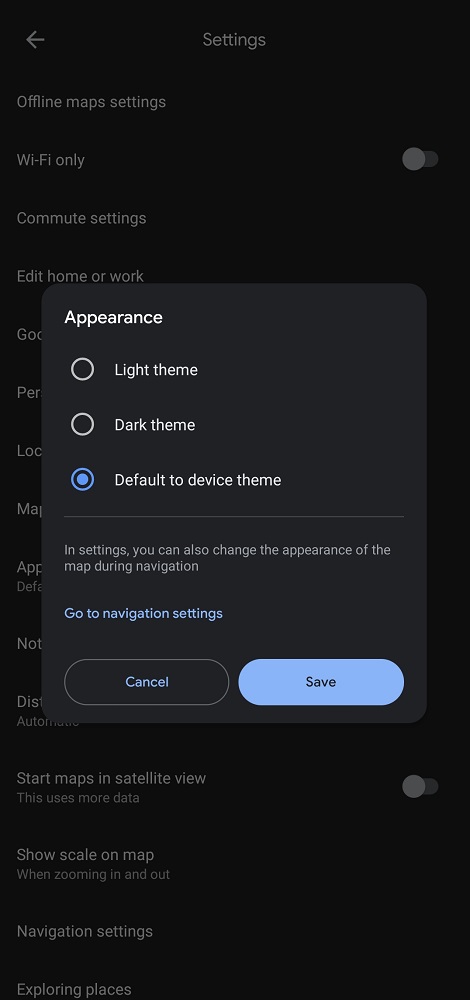This image is a vertical screenshot featuring a settings interface from an unidentified application, against a solid black background. Dominating the upper section of the screen is a pop-up window with the heading "Appearance." This pop-up obstructs much of the background, but the visible background content includes various settings options such as "Settings," "Offline Maps Settings," "Wi-Fi Only," "Commute Settings," and "Edit Home or Work." 

The pop-up window offers theme customization options: "Light Theme," "Dark Theme," and "Default to Device Theme," with the last option currently selected. Additional instructions within the pop-up indicate that map appearance can also be changed during navigation by accessing "Navigation Settings." Two buttons labelled "Cancel" and "Save" are displayed at the bottom of this window.

The partially obscured background further contains options like "Start Maps in Satellite View" with a slider button set to off, a notice about increased data usage, and the option "Show Scale on Map when zooming in and out." There are no illustrative or photographic elements accompanying the text, resulting in a plain textual display without any people, animals, birds, plants, flowers, trees, automobiles, or airplanes.